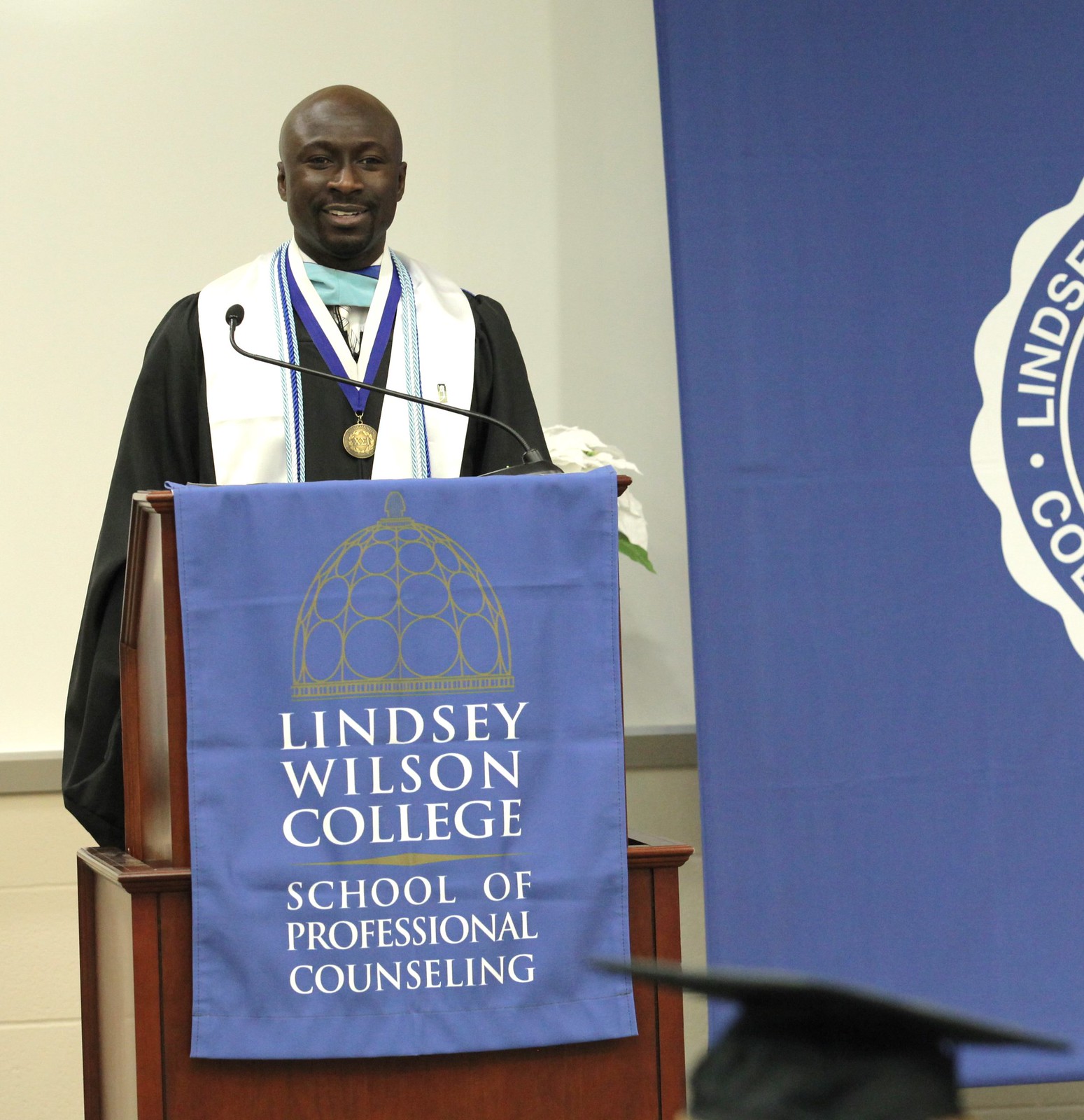The photograph captures a black man standing behind a wooden podium, delivering a speech. He is dressed in black graduation robes with white accents and is adorned with a gold-colored medal on a ribbon that is blue on the bottom half and white on the top half. The man is bald with a beard that frames his lips and chin. A microphone extends from the right side of the podium to the left, positioned in front of him. Hanging from the front of the podium is a blue banner featuring a golden dome above the text "Lindsey Wilson College School of Professional Counseling." To the right, a similar blue banner hangs, although partially cut from view, with a visible segment reading "Lindsey College." Visible in the bottom right corner of the image is the out-of-focus mortarboard cap of an audience member, suggesting that the man is addressing a graduation ceremony.